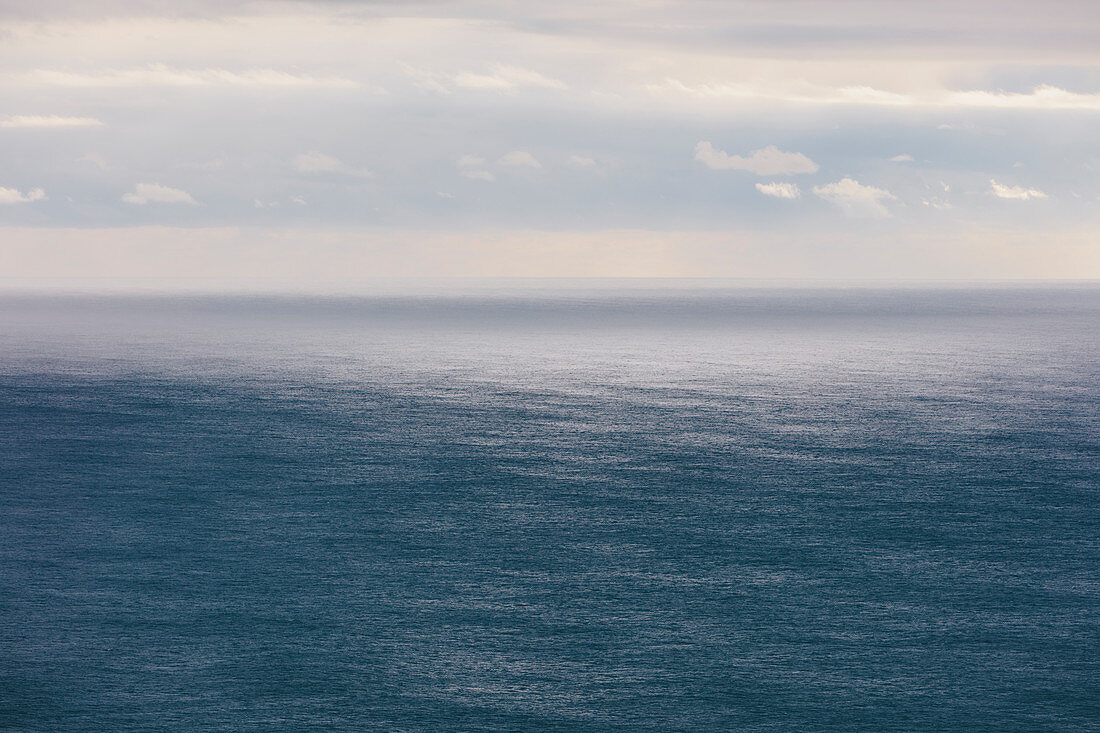The photograph captures a broad, tranquil expanse of dark blue water, likely a sea or ocean, with a seamless blend of natural light reflections. The calm surface is punctuated by large, rolling waves, suggesting the shot was taken from a boat rather than the shore, as there is no visible surf. The horizon showcases a striking contrast where the water meets a luminous, almost white reflection of light. Above this line, the sky transitions from a grayish-blue expanse, speckled with layers of both white and light gray clouds, to pockets of denser, darker clouds. The overall palette of the image spans shades of blue and gray, contributing to a serene and peaceful atmosphere. The image is outdoors, in full color, and was likely captured during a cloudy day, presenting a realistic and unembellished scene devoid of any animals, people, or identifiable landmarks. The photograph is a horizontally rectangular, borderless frame with the top third dominated by sky and clouds, reinforcing the vast, open tranquility of the seascape.